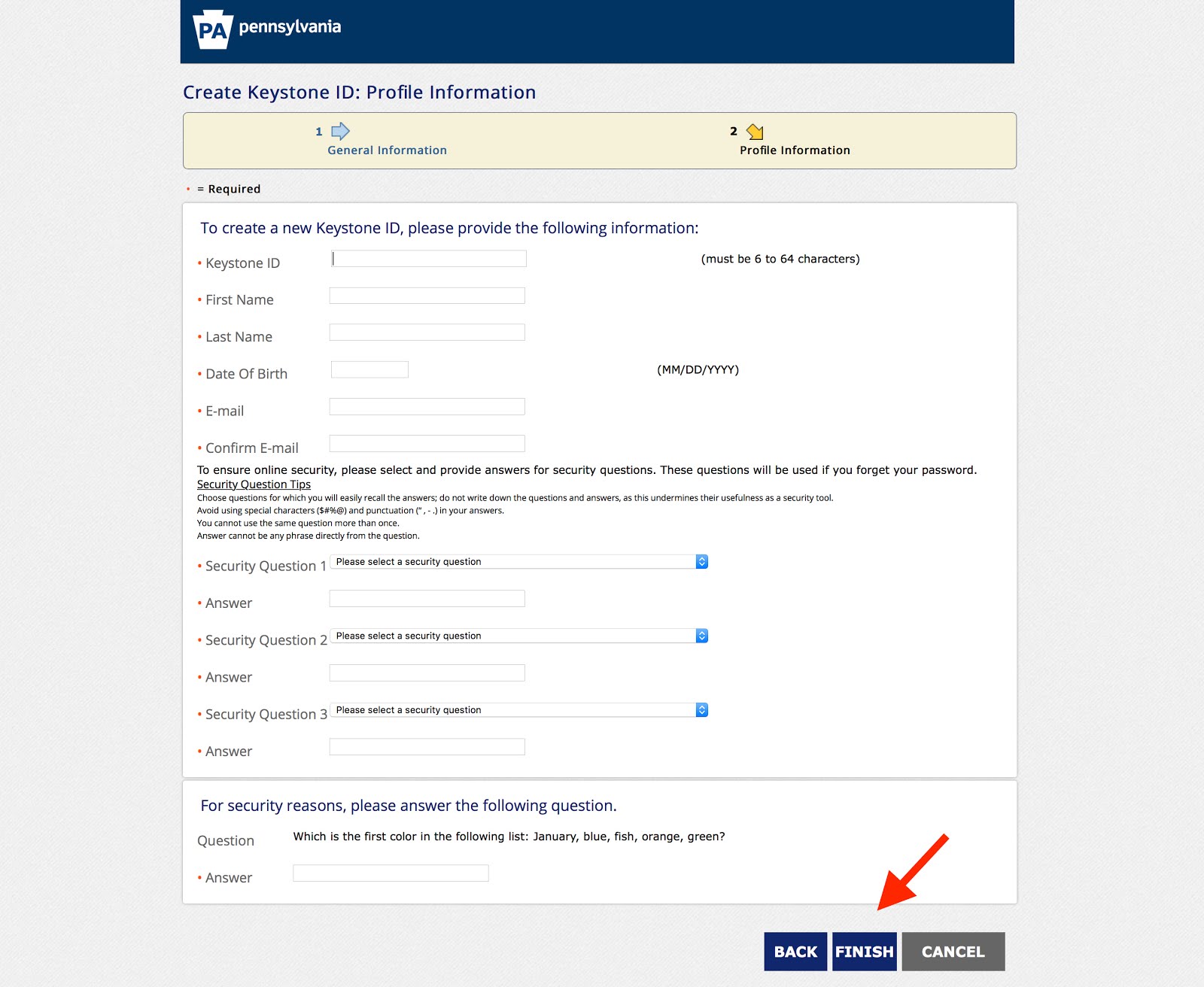The image showcases a Pennsylvania government website or application interface geared towards creating a Keystone ID profile. The official PA logo, housed within a keystone shape, is prominently displayed on a dark blue header bar. Beneath this, the title "Create Keystone ID Profile Information" is clearly written. 

The process is divided into two steps, indicated by color-coded arrows: a blue arrow pointing right labeled "General Information" for step one, and a yellow arrow pointing downward and to the right for step two, labeled "Profile Information".

A large white section below outlines the required inputs to create a new Keystone ID. Users must provide their Keystone ID (which must be between six to sixty-four characters), first name, last name, and date of birth (formatted as MM/DD/YYYY). Each of these fields is marked with a red asterisk, signifying that they are mandatory. 

Additionally, users must enter their email and confirm it, followed by selecting and answering three security questions from dropdown options. The form also includes a unique security question at the bottom: "What's the first color in the following list: January, blue, fish, orange, green?"

The form concludes with three buttons in the bottom right-hand corner labeled "Back," "Finish," and "Cancel" from left to right. The "Back" and "Finish" buttons are blue, while the "Cancel" button is gray. A red arrow points downward at the "Finish" button, drawing attention to it.